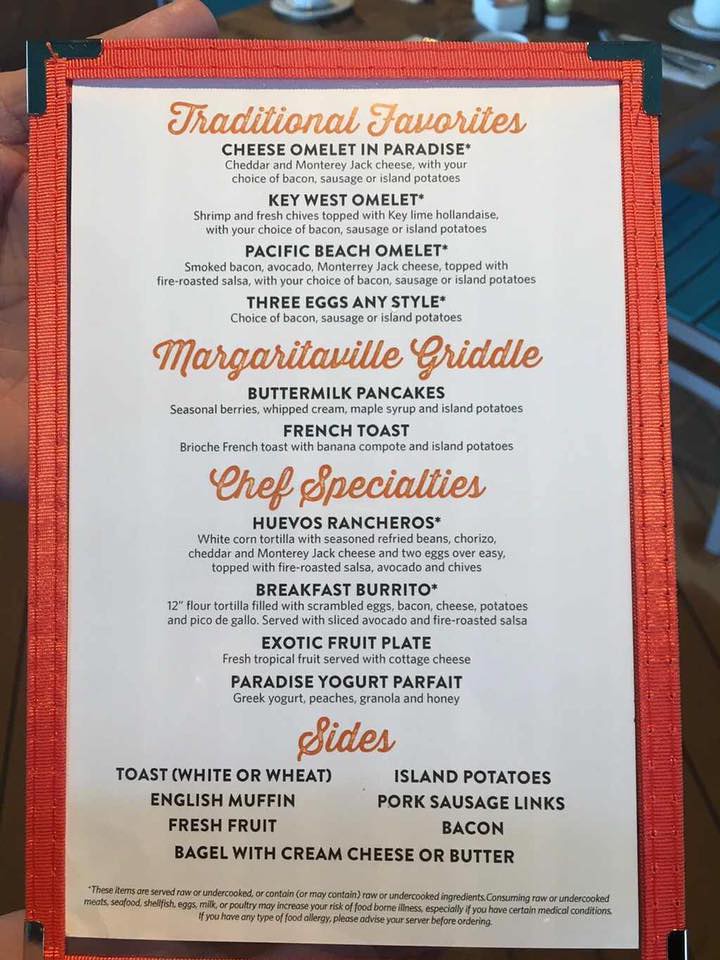This photograph captures a vibrant and well-organized restaurant menu, rich with details and thoughtful touches. The title "Traditional Favorites" is prominently displayed at the top in elegant, orange cursive, setting a warm and inviting tone, which is consistently reflected throughout the menu.

The menu features a variety of breakfast delights, starting with the "Cheese Omelet in Paradise," which boasts a delectable combination of cheddar and Monterey Jack cheese, paired with your choice of bacon, sausage, or island potatoes. Other enticing omelets include the "Key West Omelet" and the "Pacific Beach Omelet," along with a simple "Three Eggs, Any Style" option for those who prefer a classic breakfast.

Under the "Margaritaville Griddle" section, patrons can find fluffy buttermilk pancakes and sumptuous French toast, ideal for satisfying any sweet tooth. The "Chef's Specialties" offer unique dishes such as "Huevos Rancheros" and a hearty "Breakfast Burrito," ensuring there is something for everyone. An "Exotic Fruit Plate" and "Paradise Yogurt Parfait" cater to those seeking lighter fare.

The "Sides" category, also highlighted in the same distinctive orange cursive, offers a variety of accompaniments, including white or wheat toast, English muffins, fresh fruit, bagels with cream cheese or butter, island potatoes, pork sausage links, and bacon.

Each section of the menu is bordered by an orange fabric trim, which complements the cursive headings and brings a cohesive, tropical theme to the overall design. Below each item, ingredients and options are clearly listed in bold black text, ensuring clarity and helping customers make informed choices.

At the very bottom of the menu, a disclaimer addresses potential food safety concerns, stating, "These items are served raw or undercooked or may contain raw or undercooked ingredients. Consuming raw or undercooked meat, seafood, shellfish, eggs, milk, or poultry may increase your risk of foodborne illness, especially if you have certain medical conditions. If you have any type of food allergy, please advise your server before ordering."

Overall, this well-crafted menu not only highlights the restaurant's diverse offerings but also showcases a thoughtful and cohesive design that enhances the dining experience.